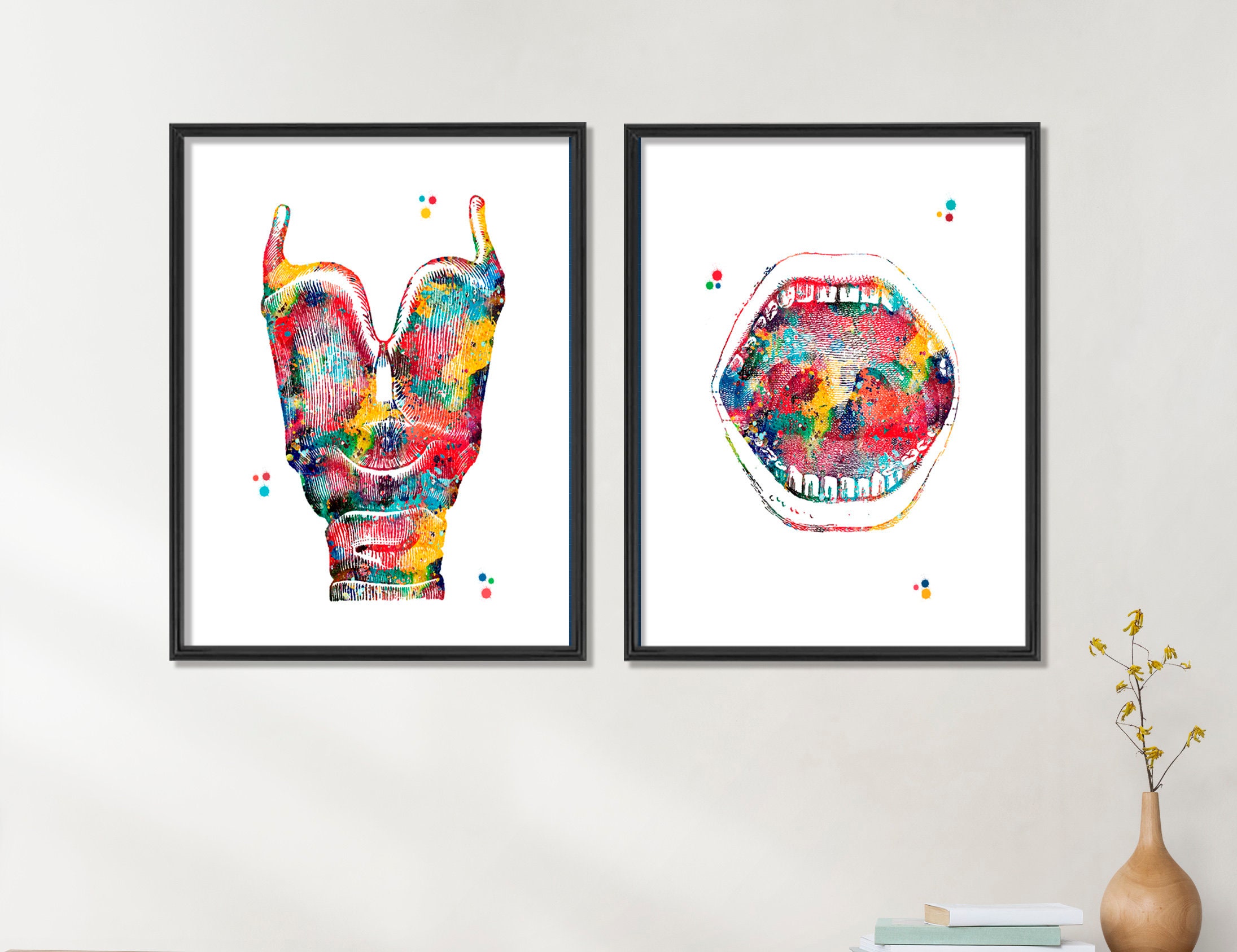On a white wall, two black-framed, colorful abstract artworks are displayed. The left piece is an enigmatic painting that could resemble either a top garment or a section of a spinal column, characterized by a curving form with segmented ridges and a vibrant mosaic of red, blue, yellow, and green hues. Surrounding the main object, tiny colored circles add to the vivid composition. The right artwork portrays a wide-open mouth with rows of perfect teeth, filled with a rainbow of colors, creating an impression of gummy bears or a watercolor mosaic. Below the framed pictures, a desk is partially visible, adorned with a plant and stacked books, adding context to the abstract display.